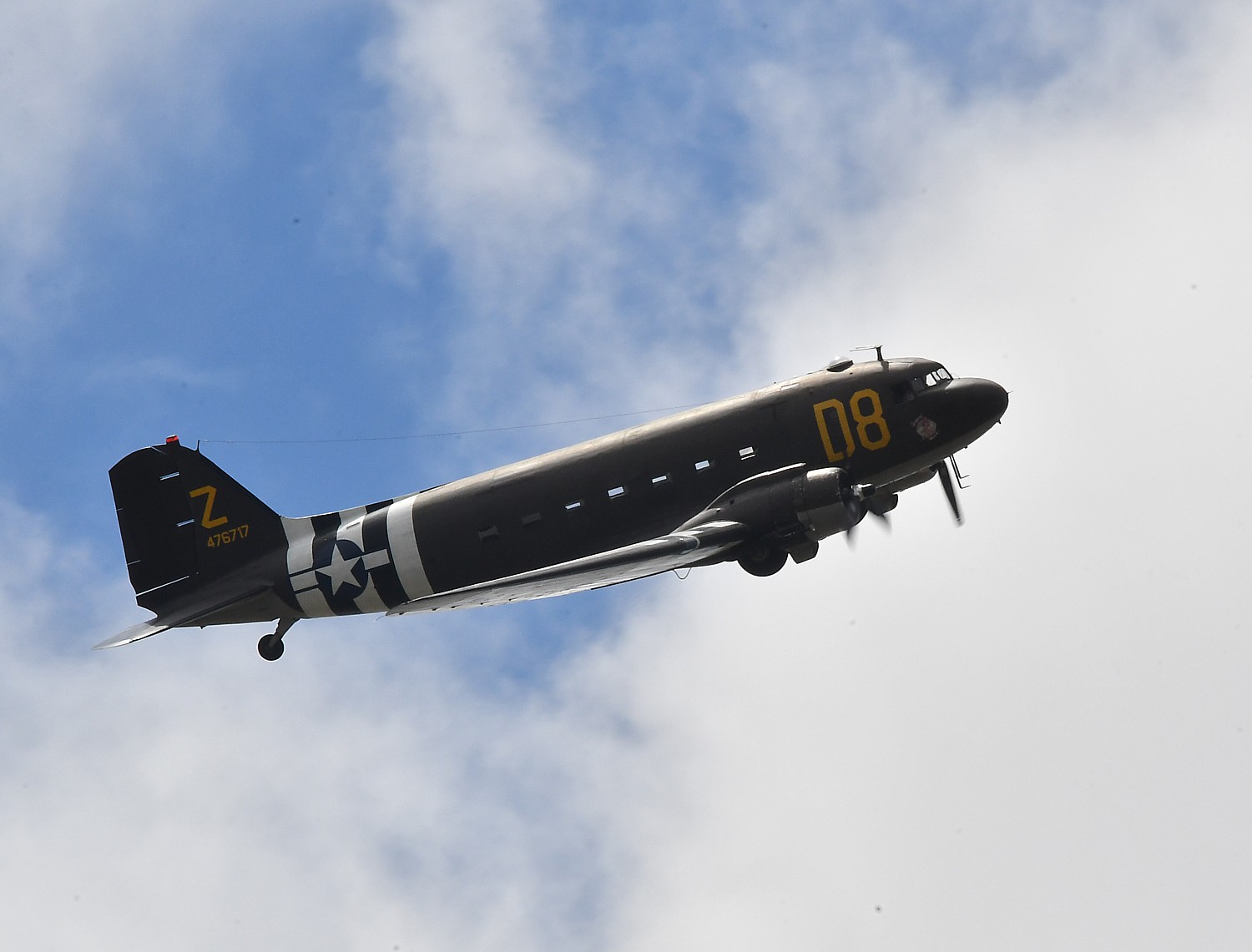The image portrays an old-fashioned fighter plane, depicted in landscape orientation, heading towards the right and angled upwards, as if ascending. The aircraft has a distinctive, rounded nose and a small, vertical cockpit window, though no pilots are visible. The plane's body is primarily dark brown, almost black, featuring black and white stripes with a prominent star near the tail. Further details include the yellow letters "D8" near the cockpit and a large yellow "Z" on the tail, accompanied by the numbers "476717." Thin wires are faintly visible along the plane's body. The propeller is actively spinning, and the scene is set against a bright blue sky dotted with fluffy clouds, suggesting a clear, sunny day.